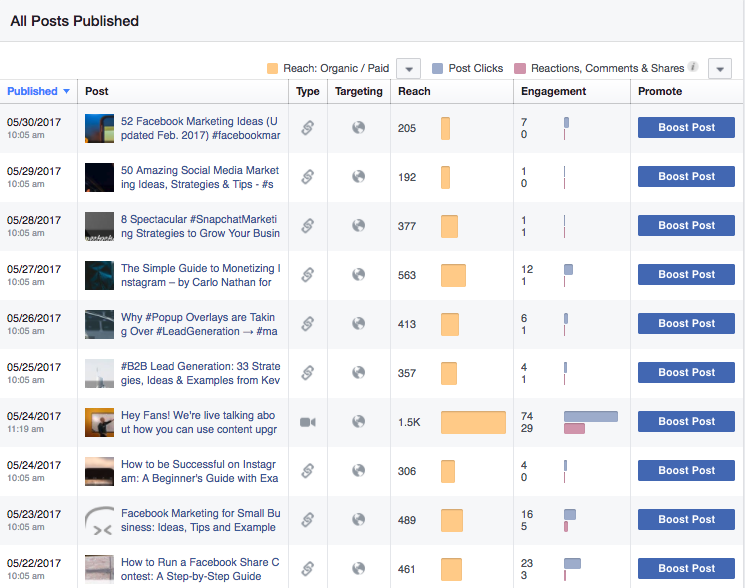This image displays a screenshot of a webpage showcasing a list of published posts, likely from a social media management tool or content management system. At the top, a gray rectangular banner stretches across the page, labeled "All Posts Published." Below this banner, the interface resembles a spreadsheet, with several columns detailing different aspects of each post.

The first column is titled "Published," with the label in blue text. This column lists the publication dates of each post, all falling within May 2017, though with varying specific dates.

The next column features a thumbnail image associated with each post, followed by a brief snippet of the post's content. Users likely need to click on these snippets to view the full posts.

To the right, there is a "Type" column indicating the format of each post. One entry is specified as a video, while others are simple image posts.

The following column is labeled "Targeting," symbolized by a globe icon for each entry, suggesting that these posts are public and globally targeted.

Next, the "Reach" column demonstrates the number of individuals each post has reached, accompanied by horizontal bar graphs illustrating this reach visually.

Adjacent to this is the "Engagement" column, showing varying numbers that likely represent likes, comments, shares, or interactions, with corresponding bar graphs beneath these figures.

Finally, in the "Promote" column, there are blue buttons labeled "Boost Post" beside each entry, offering the option to enhance the posts' visibility through paid promotion.